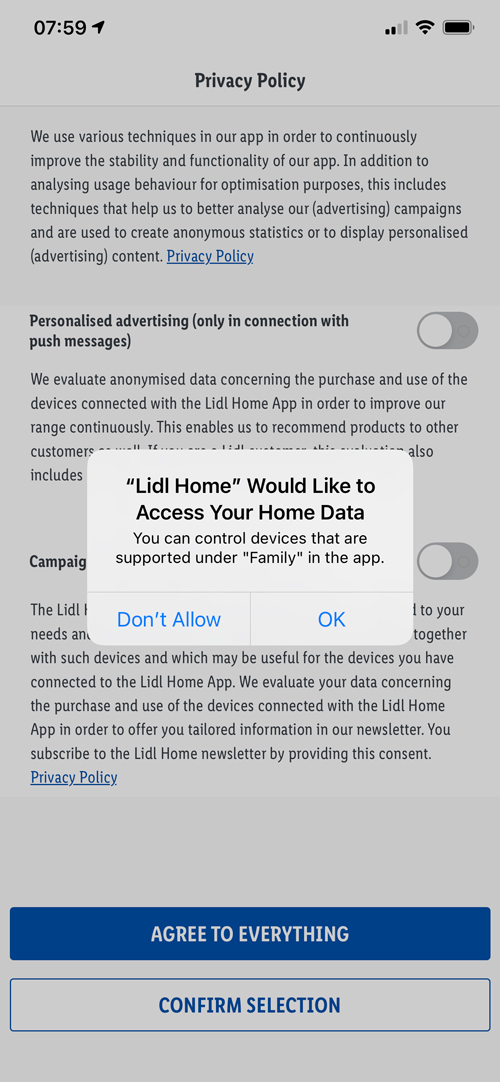This detailed caption describes a screenshot from a person's cell phone, highlighting various on-screen elements at 7:59. At the top, icons indicate two bars of cellular coverage, full Wi-Fi, and a fully charged battery. The background is slightly grayed out, and the focal point is a prominent white pop-up window in the center. This pop-up, from the LIDL Home app, requests access to the user's home data to control supported devices. The user has the options to "Don't allow" or "OK."

The pop-up partially obscures text that discusses the app's privacy policy and its methods for enhancing app stability and functionality. It mentions that data is anonymized for optimizing usage patterns, analyzing advertising campaigns, and generating anonymous statistics or personalized content. Personalized advertising is linked with push notifications, and the data from connected devices are analyzed to improve product recommendations continually.

Underneath the obscuring pop-up, partially visible text explains that such device evaluations help tailor newsletter content to the user's connected devices. By subscribing to the LIDL Home newsletter, the user consents to these terms, which are reiterated in the visible privacy policy statements. The user has not interacted with any options yet. At the bottom of the screen, two buttons read "Agree to everything" and "Confirm selection."